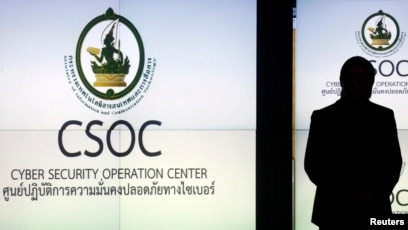The image appears to be a detailed wall poster or possibly a screenshot from a video. The central feature is a large white sign that dominates the left-hand side, taking up about two-thirds of the width. At the top of the sign, there is an oval logo with a green outline, containing a humanoid figure possibly of oriental origin, holding a gold or yellow bar in one hand. The figure's other hand is raised, possibly holding a dagger or a similar object. Beneath this logo, the poster prominently displays "CSOC" in bold black letters, which stands for "Cyber Security Operations Center." Below this, the text continues in what is likely Arabic or another Middle Eastern language. 

On the right side of the image, a vertical black strip separates the main poster from a smaller section. In front of this black strip stands the silhouette of a man, and nearby, in the lower right corner, the word "Rutgers" is visible in small white print.

Overall, the scene includes repeating elements of the CSOC logo and text, creating a sense of continuity across the poster.